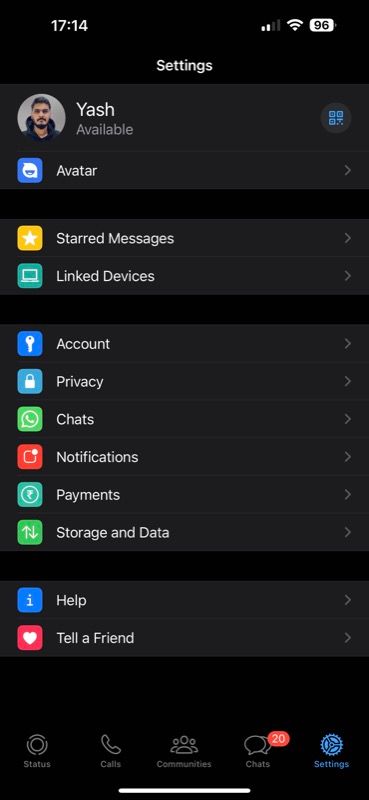This image is a screenshot taken from a cell phone displaying a settings menu, possibly from an Android device. The background is composed of varying shades of black, with slightly lighter black tones used to differentiate text and icons. The time is shown in military format (24-hour time) as 17:14. 

In the top-right corner of the screen, the phone's status is visible, indicating two bars of cellular signal strength and a Wi-Fi connection. The battery icon shows a charge level of 96%.

The top section of the screenshot shows the title "Settings," followed by a thumbnail image of a man named Yash (capital Y-A-S-H). Beneath his photograph is the status "Available." 

The settings menu lists several options in order: 
- Starred Messages
- Linked Devices
- Account
- Privacy
- Chats
- Notifications
- Payments
- Storage and Data
- Help
- Tell a Friend 

Each option is likely represented by an accompanying icon, commonly seen in Android settings interfaces.